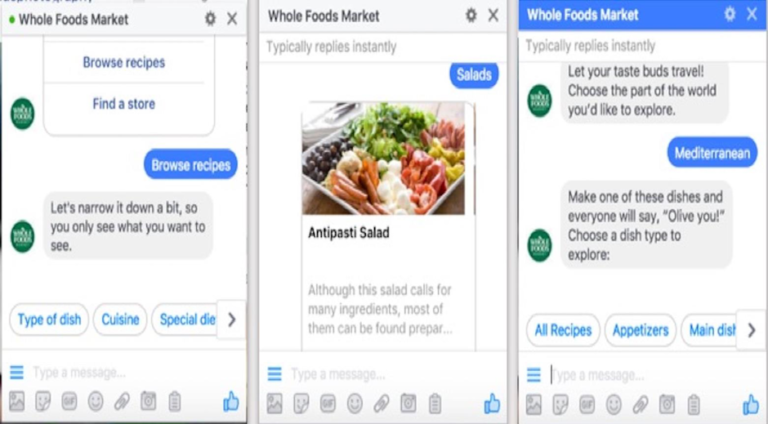The image depicts a user interface on the Whole Foods Market website, where a chatbot is assisting someone in meal preparation. The user is engaged in an interactive process of refining their recipe search, initially opting to browse for general recipes, then narrowing down to salads, and finally focusing on Mediterranean salads. One of the prominent screens showcases an appetizing antipasti salad, complete with a vibrant image of the dish and a detailed list of ingredients. The interface encourages culinary exploration with headings like "Let your taste buds travel" and presents the option to choose different parts of the world to discover various dishes. The user inputs "Mediterranean," prompting the chatbot to filter and display relevant recipes. The system illustrates an intuitive narrowing process, where entering keywords prompts the chatbot to find and suggest matching recipes, guiding the user to select and prepare a desired dish seamlessly.